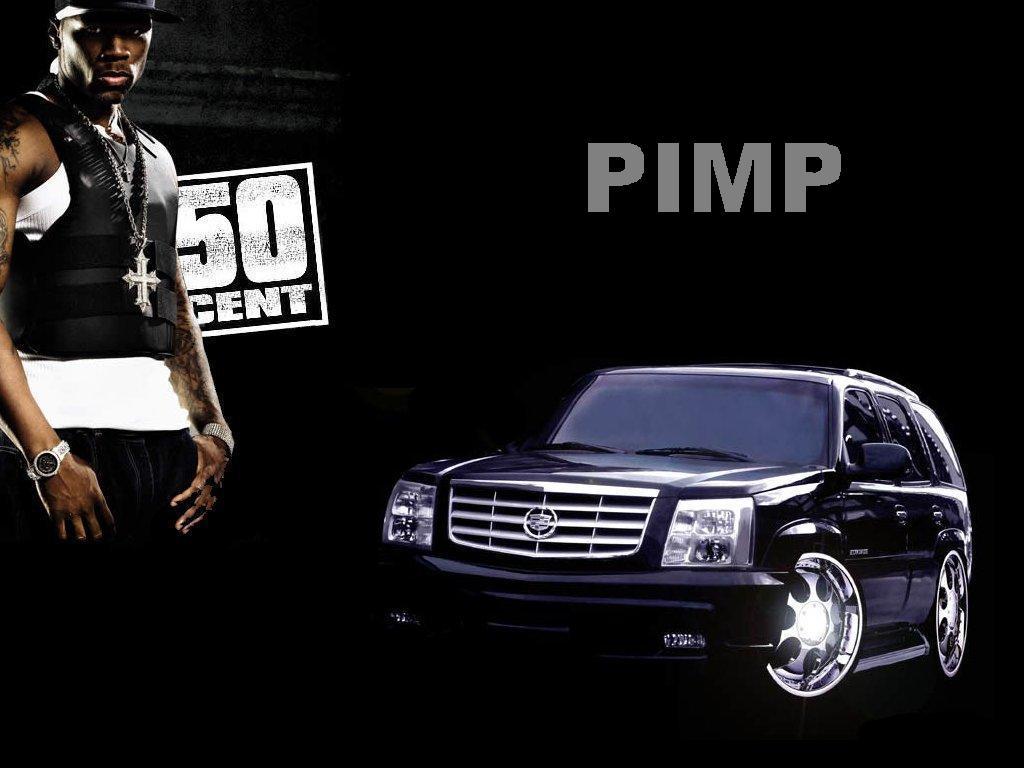The image appears to be a promotional poster featuring a split composition on a dark black background. On the left side stands the rapper 50 Cent, depicted in a stern pose while looking directly into the camera. He is wearing a black baseball cap (partly cut off in the image), a black bulletproof vest over a white tank top, and black pants. Around his neck hangs a prominent silver cross on a matching chain, and he sports two silver watches on his wrists. Behind him is a distinct 50 Cent logo in white lettering. 

On the right side of the image, the lower half features a shiny black Cadillac Escalade with silver wheels and a silver grille, exhibiting a glossy finish with its wheels slightly turned to the left. Above the images, in large gray uppercase letters, the word "PIMP" is displayed. The visual elements and careful detailing suggest this could be an album cover or promotional material.